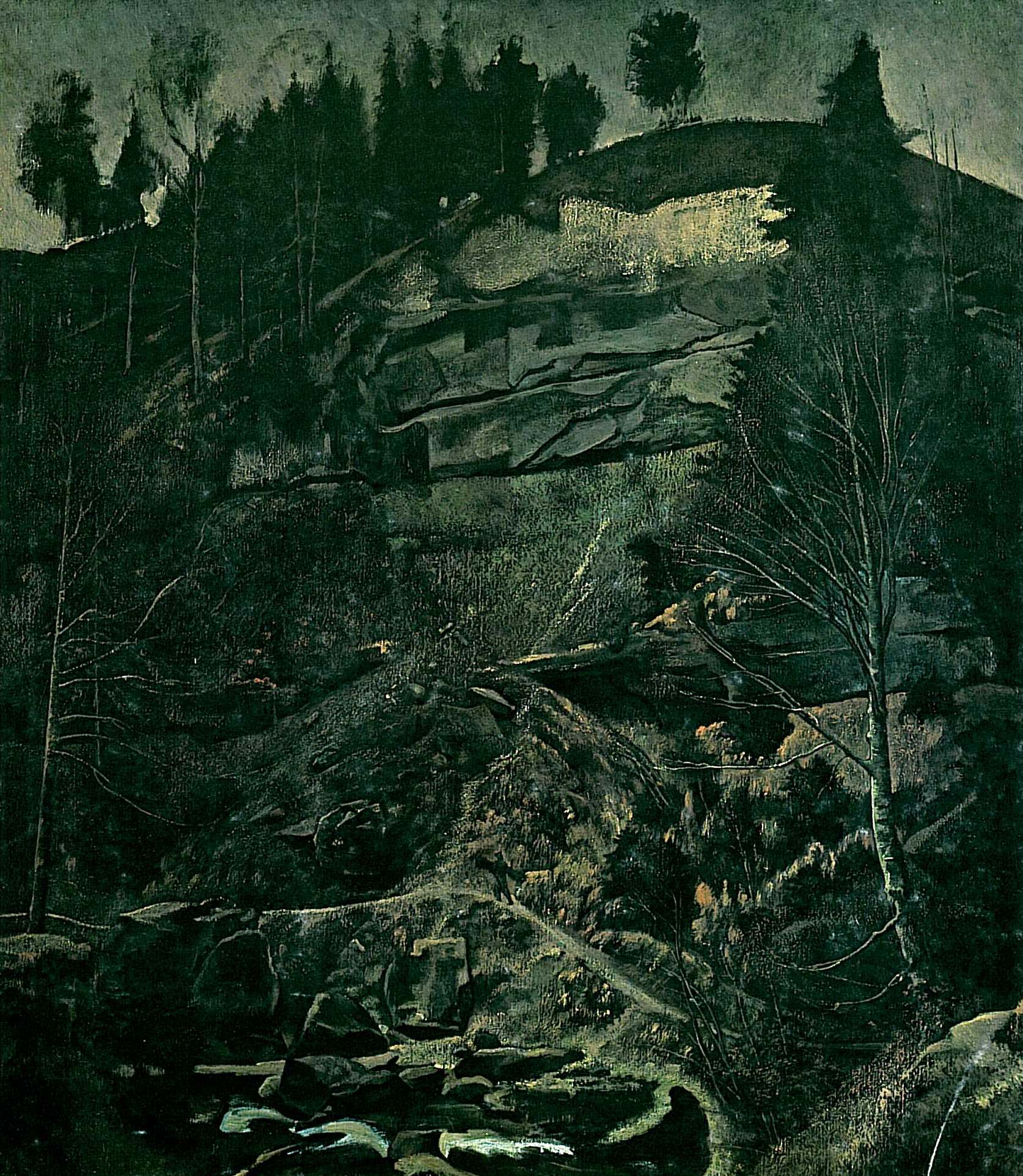The image appears to be a dark, eerie painting of a desolate hillside scene. Dominated by dark green, black, and gray tones, the artwork creates a spooky atmosphere. The hillside itself is steep and rocky, with bare, leafless trees scattered on both sides—one prominent tree to the right and a similar one to the left. In the bottom section, there is a body of water, flanked by more rocks. The background showcases larger, taller trees, possibly pine trees, which cast dark, looming silhouettes against a dim, almost indistinguishable sky. The entire composition has a bleak and shadowy feel, invoking an unsettling mood as the dark colors blend intricately into one another. There are no human figures or any text within the image, further enhancing its lonely, foreboding impression. The scene seems to capture an outdoor setting, perhaps in the middle of the day, though the pervasive darkness cloaks it in a haunting light.